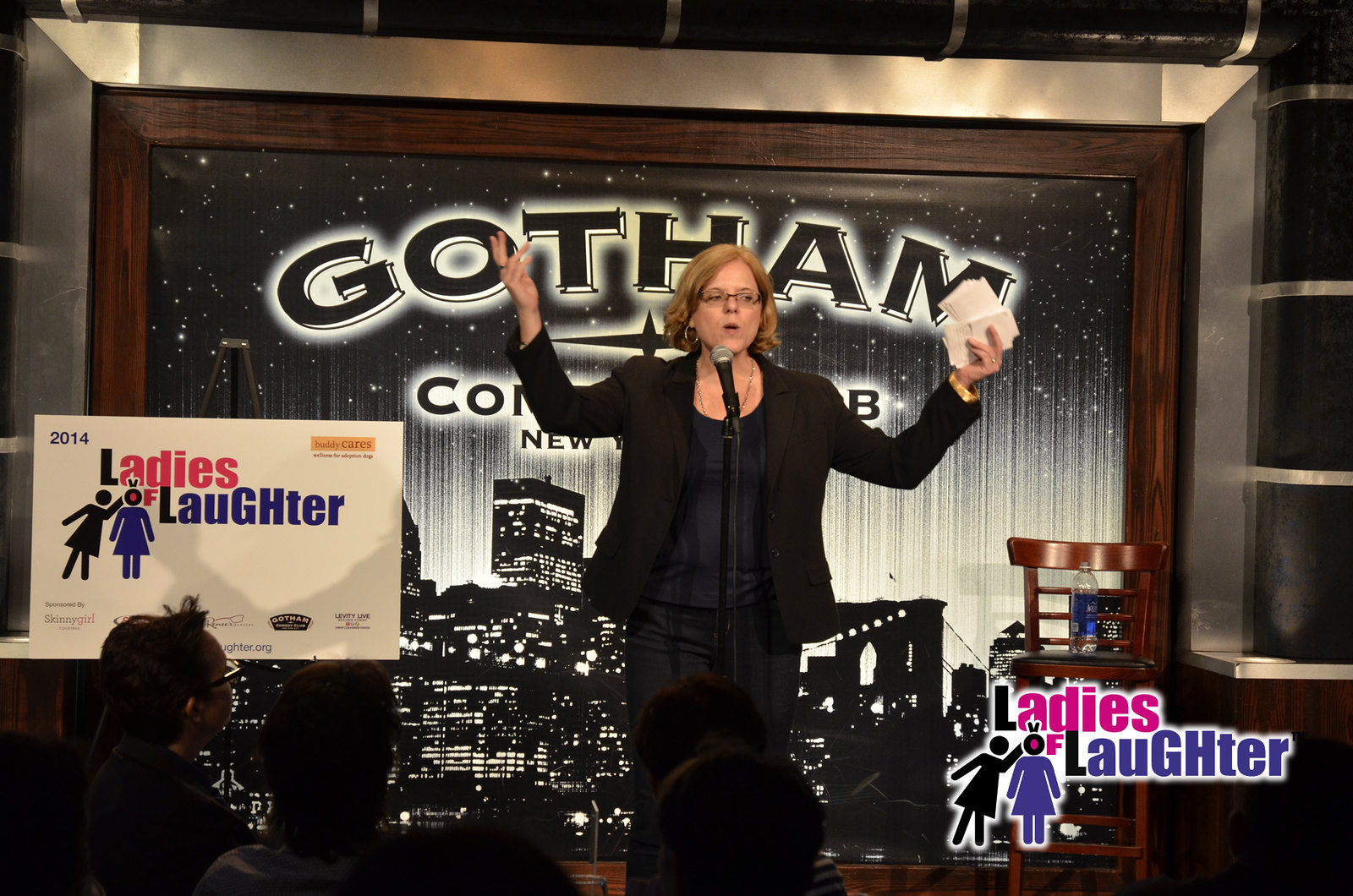The image depicts a woman performing stand-up comedy in front of a backdrop featuring the Gotham Comedy Club banner in New York City. She is dressed in a black outfit, including a black jacket, black shirt, and black pants. Her short blonde hair is complemented by glasses, and she holds a few 3x5 cue cards in her right hand. The backdrop showcases a black-and-white view of the New York skyline, including a bridge, and is partially obscured by the woman. Above her, the large text "Gotham" is followed by smaller text reading "Comedy Club" and "New York." To the left, there is a smaller white poster with "2014 Ladies of Laughter," featuring a woman in a blue dress and another in a black dress, with one of their heads forming the "O" in "of." This logo also appears in the lower right corner of the image, superimposed in black, pink, and purple text. The audience's silhouettes are visible along the bottom edge of the photo, adding to the lively atmosphere of the comedy performance.